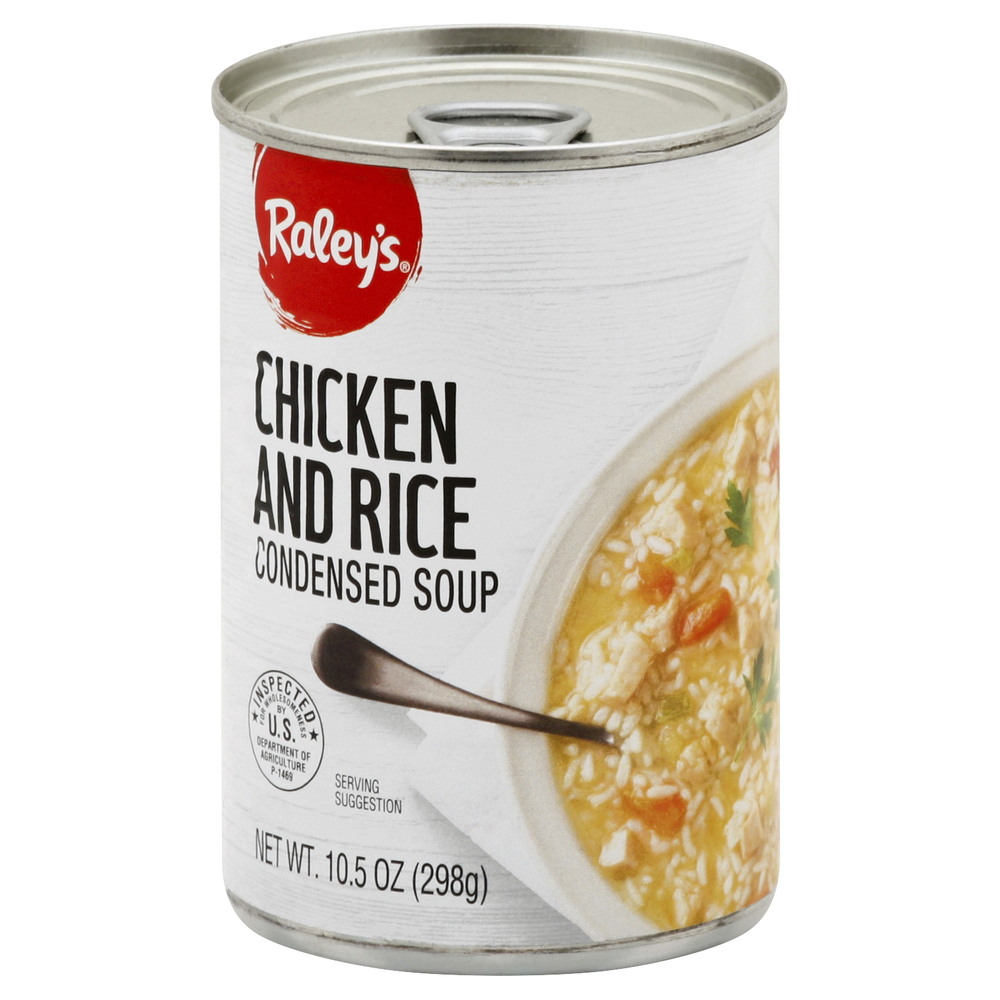A close-up image features a small cylindrical metal can of Rayleigh's Chicken and Rice Condensed Soup, set against a white background. The can is made of gray metal with a rim at both the top and bottom, and it has a gray lid that includes a pull-tab opening. The can's label spans the entire front, with a white background and detailed illustrations. Prominently displayed on the label is a white ceramic bowl filled with chicken and rice soup, complete with visible pieces of chicken, orange carrot slices, green herbs like parsley or basil, and white rice. A metal spoon is sticking out of the bowl. Above the image of the soup, there is a red circular logo with "Rayleigh's" in white text, followed by "Chicken and Rice Condensed Soup" in black text. Additional text on the label mentions "Inspected by U.S. Department of Agriculture," "Serving suggestion," and "Net weight: 10.5 ounces, 298 grams." The can is slightly angled in the photograph, offering a clear view of the soup and text on the label. The colors visible include red, white, black, silver, orange, green, light brown, and off-white.